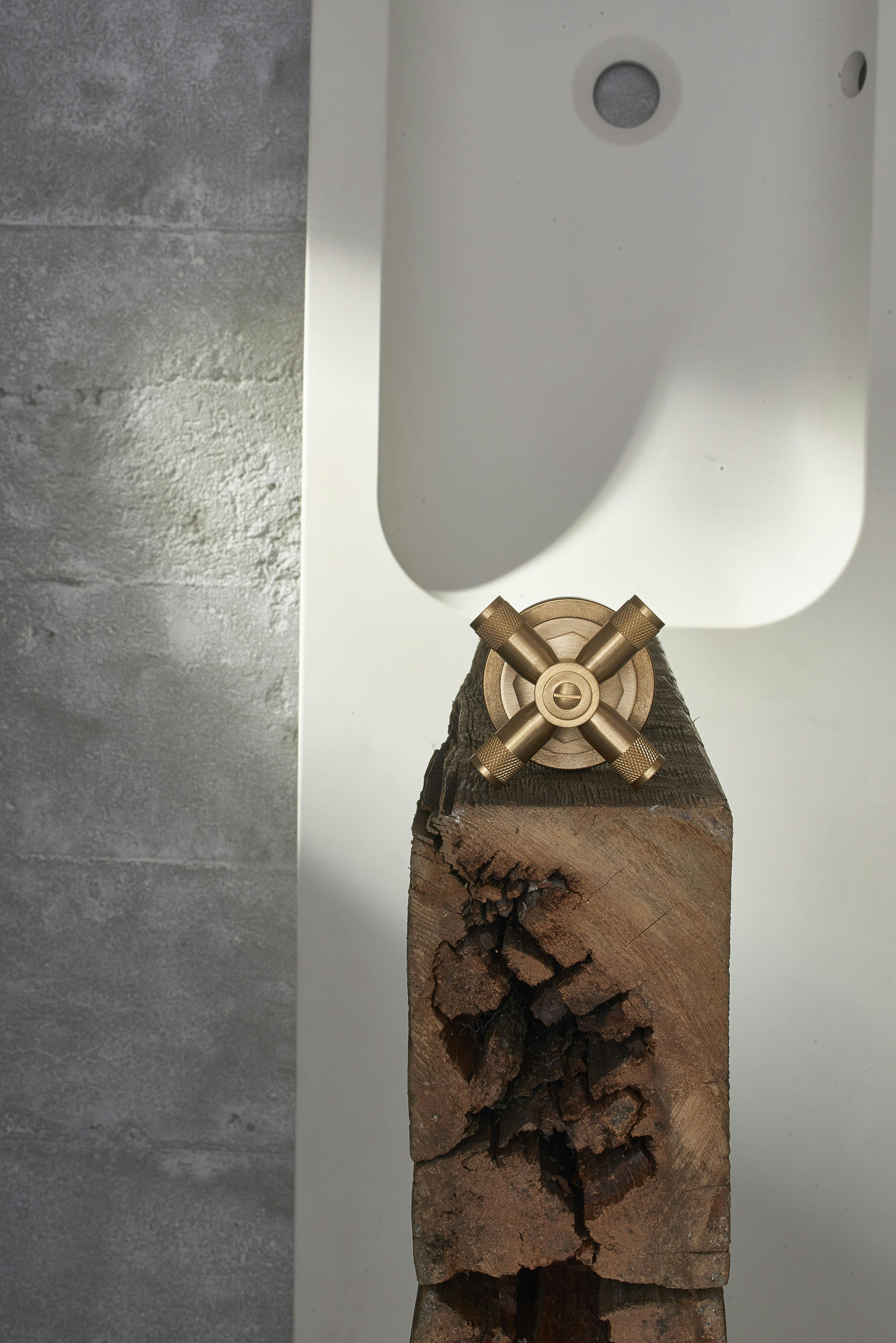This is a top-down image of an indoor setting featuring a white porcelain sink or tub placed on a backdrop of large gray concrete tiles or slabs. The white porcelain piece has a bowl in the center with a couple of circular holes—one at the bottom presumably for drainage, and another on the right-hand side that acts as a spillway. A standout element in the image is a wooden block situated at the bottom center, appearing to have weathered, darkened wood grain that shows signs of age. This wooden block holds a brass fixture on top with an X-like pattern, suggesting the design of an old-fashioned spigot or a hose connector. The brass handle, with its four extensions, hints at an artisanal touch, further enriching the rustic aesthetic of the scene. The photograph, taken during the daytime, focuses on this intricate setup from an overhead perspective, capturing various hues of white, gray, brown, and bronze, which add depth and character to the overall composition.